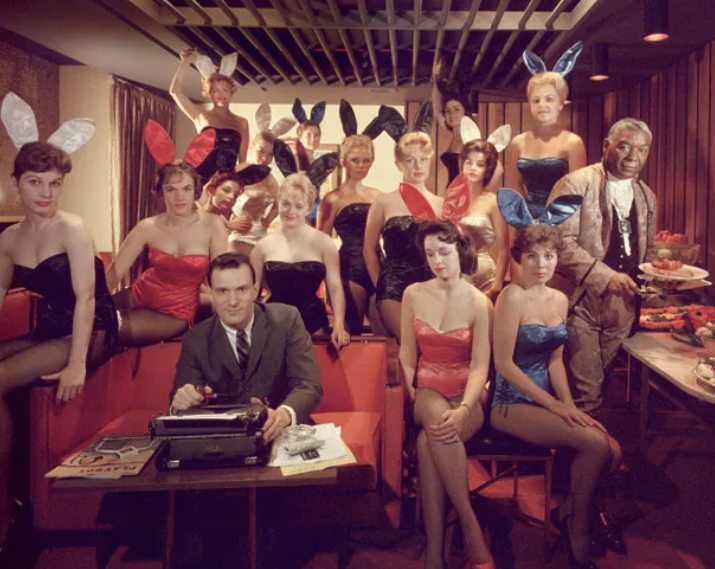In this washed-out photograph from the 50s or 60s, taken inside what appears to be Hugh Hefner's Playboy Mansion, Hugh Hefner is sitting on an orange-red couch (or bench) in an elaborate wooden-paneled room with a large curtain on the left side. He is dressed in a suit and tie, seated in front of a typewriter with his left hand resting on it and holding a pipe in his right hand. Just to his right, on a coffee table that holds the typewriter, lies a Playboy magazine. Surrounding Hefner are about a dozen Playboy bunnies wearing sleeveless, strapless bodysuits and the iconic Playboy bunny ears in various colors including white, red, black, and blue. To the far right, an African American man stands near a buffet table, dressed in an elaborate brown tuxedo with a dark vest, holding a plate of food. One woman near him is also visible. Most of the women appear to be caucasian and, while they are looking into the camera, their expressions vary and many do not look overly joyful. The setting and attire indicate a classic scene emblematic of the Playboy brand during that era.